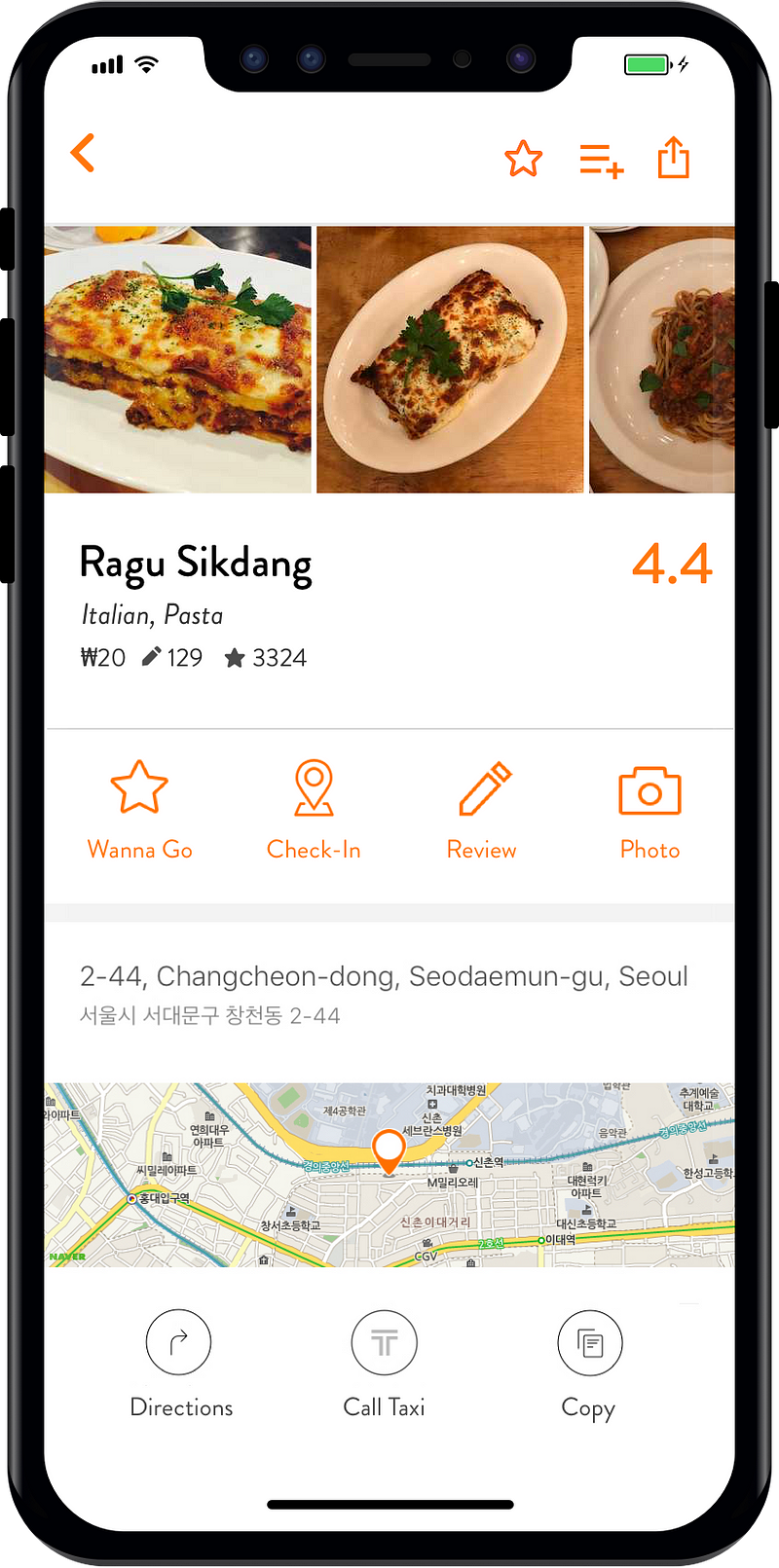The image appears to be an advertisement for a restaurant displayed on a phone screen. At the top of the screen, you can see the typical phone status indicators: four bars indicating reception strength, a Wi-Fi icon, and on the right, a green battery icon suggesting the battery is charging.

Below the status indicators, there's a white space featuring an orange arrow pointing to the left. To its right, three icons are displayed. 

Moving down, there's a section with three square images. The first image shows a dish that resembles lasagna. The second image provides a top-down view of the same lasagna dish, garnished with green herbs and served on a white oval plate. The third image is partially cut off and appears to show a noodle dish on a round white plate.

Following the images, the text "Ragu Sikdang" is displayed with a 4.4 rating next to it, indicating customer reviews. It lists the restaurant's specialties as Italian cuisine and pasta. There are also interactive icons labeled "Want to Go," "Check In," "Review," and "Photo."

The address section indicates that the restaurant is located in Seoul, Korea. Additional options provided include viewing a map, getting directions, calling a taxi, and copying the address details.